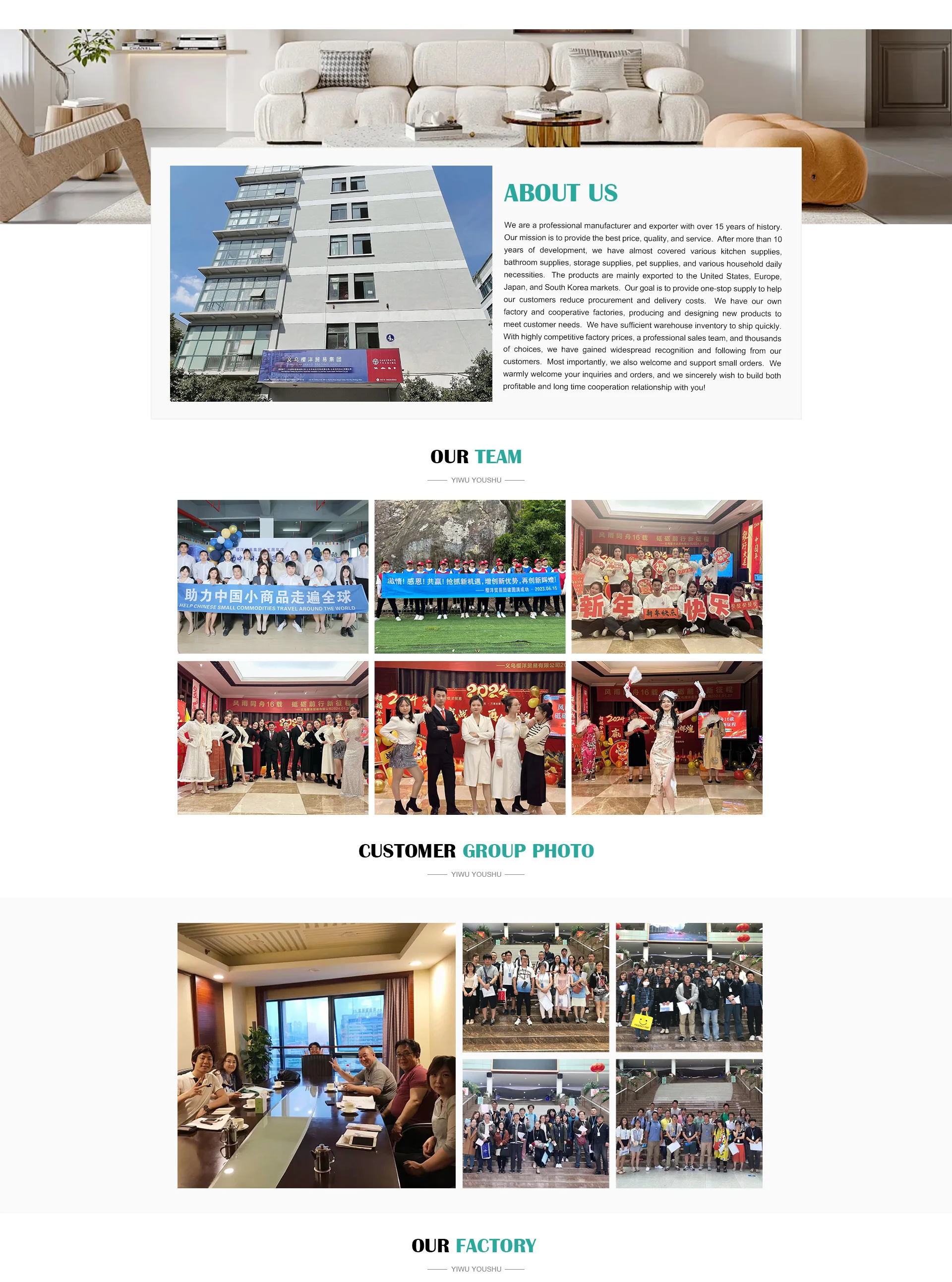In this website screenshot, the background captures a modern interior space with a grey tiled floor and a pristine white wall. A dark grey door can be seen in the upper right corner. Centrally positioned against the wall is a white, plush couch. Superimposed on this scene is a light grey rectangle. On the left side of this rectangle is a photograph of an apartment building, showcasing grey walls on the right and blue windows on the left. Adjacent to the photograph, bold teal text in all caps reads "About Us."

Beneath this header lies a comprehensive paragraph in black text detailing the company's profile. It states: "We are a professional manufacturer and exporter with over 15 years of history. Our mission is to provide the best price, quality, and service. After more than 10 years of development, we have almost covered various kitchen supplies, bathroom supplies, storage supplies, pet supplies, and various household daily necessities. The products are mainly exported to the United States, Europe, Japan, and South Korea markets. Our goal is to provide one-stop supply to help our customers reduce procurement and delivery costs. We have our own factory and cooperative facilities producing and designing new products to meet customer needs. We have sufficient warehouse inventory to ship quickly. With highly competitive factory prices, professional sales team, and thousands of choices, we have gained widespread recognition and following from our customers. Most importantly, we also welcome and support small orders. We warmly welcome your inquiries and orders, and we sincerely wish to build both profitable and long-time cooperation relationship with you."